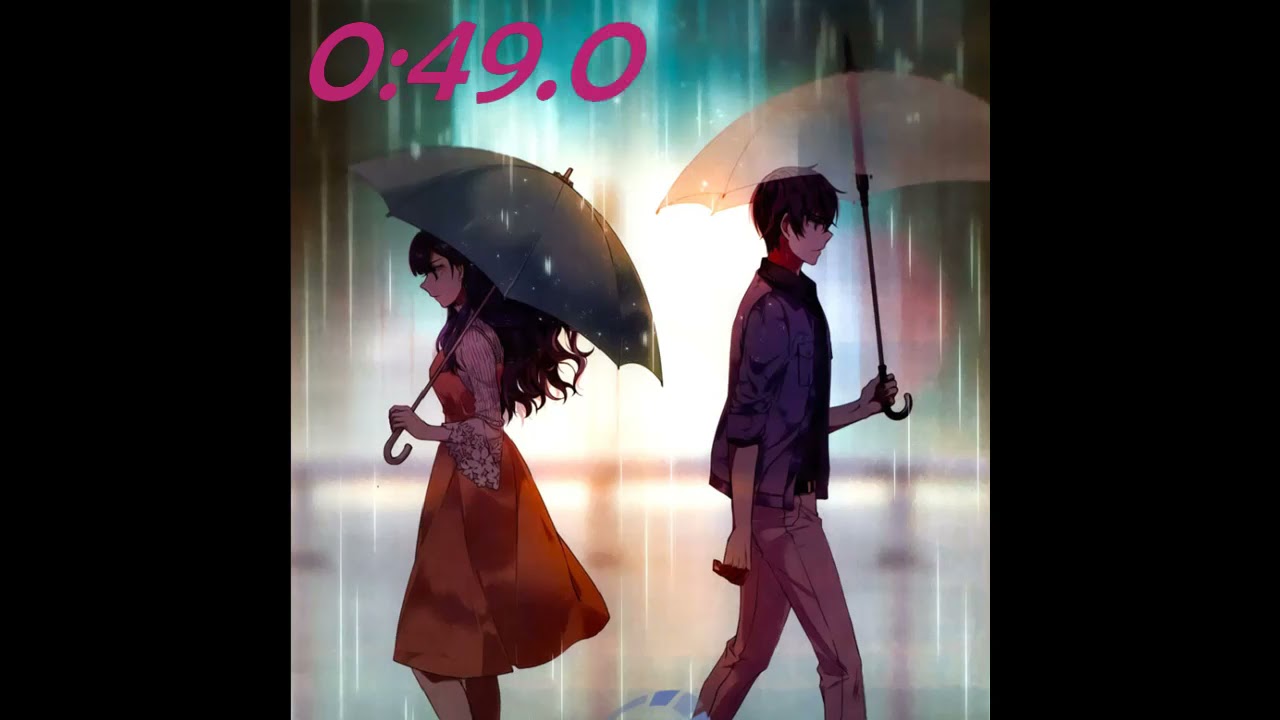This detailed anime-style illustration depicts a man and a woman walking away from each other amidst a heavy downpour, set against a dark background. The woman, with her long, wavy brown hair cascading over her shoulders, is adorned in an orange dress with white or magenta pink sleeves, and she clutches a black umbrella. In contrast, the man, with his short, dark, ear-length hair, sports a blue long-sleeve shirt and khaki pants as he holds a white, transparent umbrella. Both are positioned almost back-to-back yet moving in opposite directions, she to the left and he to the right, along what appears to be a bridge evident from the small rail guard visible in the background. The intense rainfall is suggested by the umbrellas they carry. The scene is punctuated with magenta numbers reading "0:49.0" in the upper left-hand corner, giving it a distinctive timestamp-like element, all set against a predominantly black backdrop.